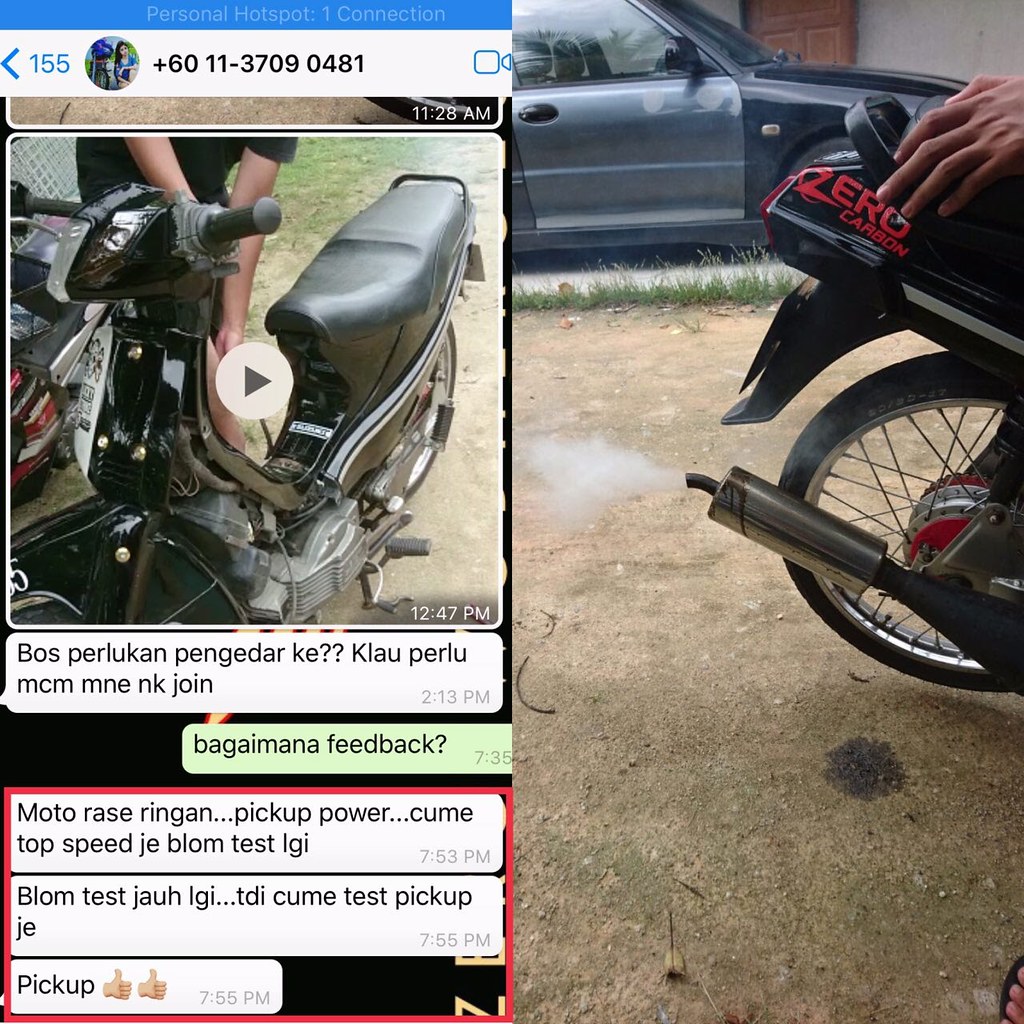The image is split into two sections. On the left is a screenshot of a text conversation in a foreign language, showing messages exchanged presumably about purchasing or picking up a motorcycle. Mixed in with the foreign text are English words and phrases such as "feedback?", "pick up power", "top speed", "test pickup", and a thumbs-up emoji. This portion also displays the time "12:47 p.m." and indicates a personal hotspot connection. 

On the right side of the image, there's a photo of a motorcycle's rear half, featuring the back tire, seat, and exhaust pipe. A hand is visibly gripping the back of the seat. The motorcycle itself appears to be black with red markings that read "zero carbon." In the background, there's a car. Notably, this car has a dark blue or black body with a light blue passenger side door. The motorcycle is parked on a driveway with a small oil spot beneath it, and the setting appears to be outdoors, possibly on a patch of dirt.